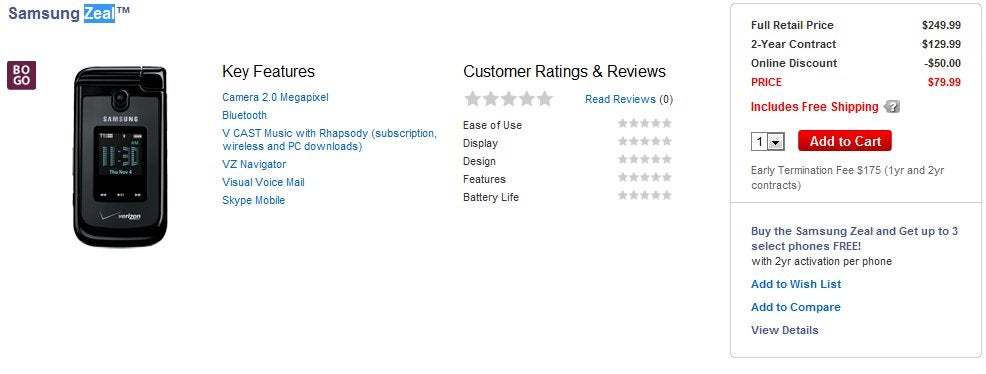Introducing the Samsung Zeal™ - A sleek, black flip phone designed for ultimate convenience. This model features vibrant blue text highlighting its key features, making it effortless for users to navigate. Underneath the product details, it indicates that there have been no customer ratings or reviews yet. The full retail price of the Samsung Zeal™ is $249.29, but with a two-year contract and an online discount of $50, it is available for just $79. This offer includes free shipping.

Customers can add this product to their cart with an early termination fee of $175 applicable. As an added incentive, purchasing the Samsung Zeal™ includes an offer to get up to three select phones for free, provided each has a two-year activation plan.

Options to add the phone to a wish list, compare it with other models, or view additional details are easily accessible. Make the Samsung Zeal™ your next phone choice for a combination of style, functionality, and exclusive savings.